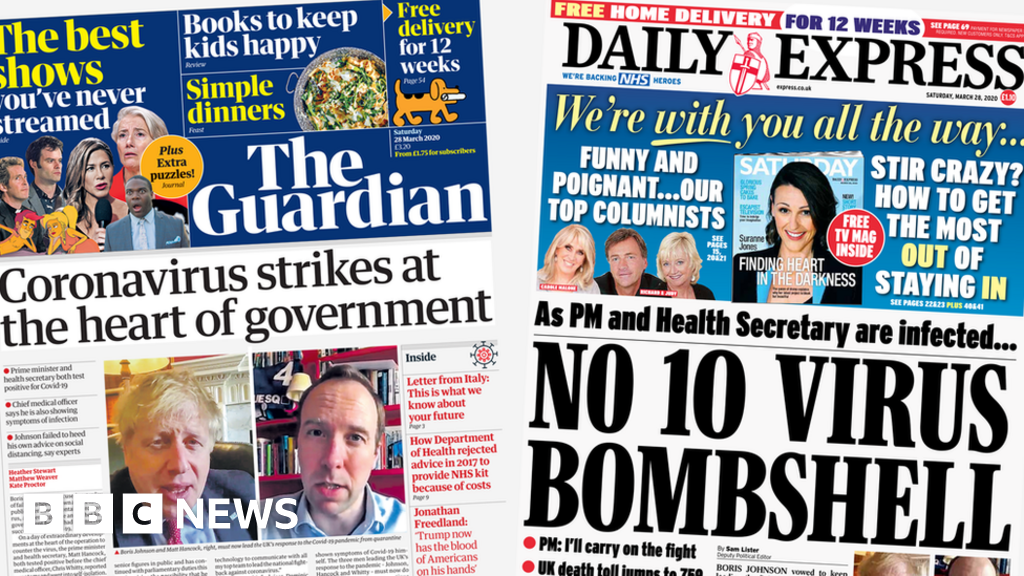Here are two detailed descriptive captions for the images of the tabloids:

1. **The Guardian Tabloid Screenshot**: The left side of the image features a screenshot of a cover from "The Guardian" tabloid. The prominent headline in yellow text declares "The Best Shows You've Ever Dreamed." Below this, in white text against a blue background, it states, "Books Keep Kids Happy." Another highlighted section in yellow reads "Simple Dinners," accompanied by an image that appears to be of a pizza. Additionally, there's a bold offer of "Free Delivery for 12 Weeks." The Guardian's leading news story addresses the coronavirus outbreak with the headline, "Coronavirus Strikes at the Heart of Government." The tabloid prominently features its branding, with the name "The Guardian" clearly displayed.

2. **Daily Express Tabloid Screenshot**: The right side of the image showcases a cover from the "Daily Express" tabloid. At the top, a red banner announces "Free Home Delivery for 12 Weeks," with the phrase "For 12 Weeks" highlighted in blue and the rest of the text in yellow and red. The "Daily Express" logo is displayed in black text, featuring a distinctive red crusader emblem between "Daily" and "Express." The leading stories include "We're With You All The Way," "Funny Appointment," "Our Top Columnists," and "Stir Crazy: How to Get the Most Out of Staying In." A significant headline concerning the coronavirus reads, "As PM and Health Secretary Are Infected, No 10-Virus Bombshell."